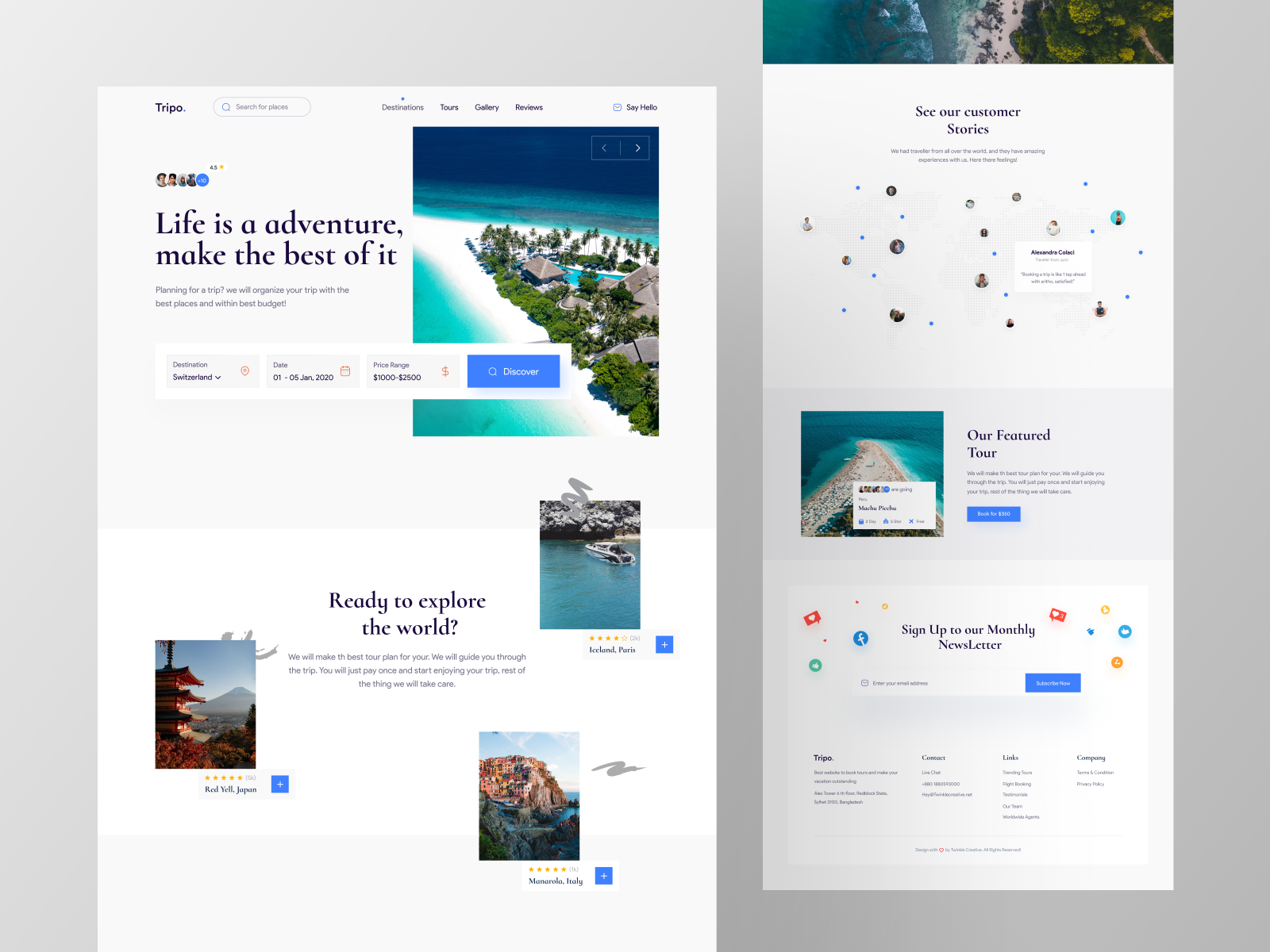This image is a detailed screenshot of the TRIPO website or app interface. At the top left corner, there's an inspiring tagline: "Life is an adventure, make the best of it." Directly to the right of this text, there's a serene photograph depicting a beach resort. This resort is nestled on a piece of land surrounded by pristine white sand, with azure blue waters encircling the sandy area. To the far right, there is an interactive bot, which likely provides user assistance.

Beneath the main beach image, there's a smaller photo featuring a boat on crystal-clear water, accompanied by the phrase, "Ready to explore the world." On the left side of the screen, there's another smaller image showcasing a traditional building in Japan, giving a hint of the diverse travel destinations offered by TRIPO. In the bottom right corner, yet another picture features a cityscape perched dramatically atop a cliffside, suggesting adventurous and picturesque city destinations.

Spanning the top of the beach photo, there's a navigation bar that includes several drop-down options: one for selecting a travel destination, another for choosing travel dates, and a third for setting a price range. The flow of the interface culminates in a prominent blue button labeled "Discover," inviting users to start their travel planning journey.